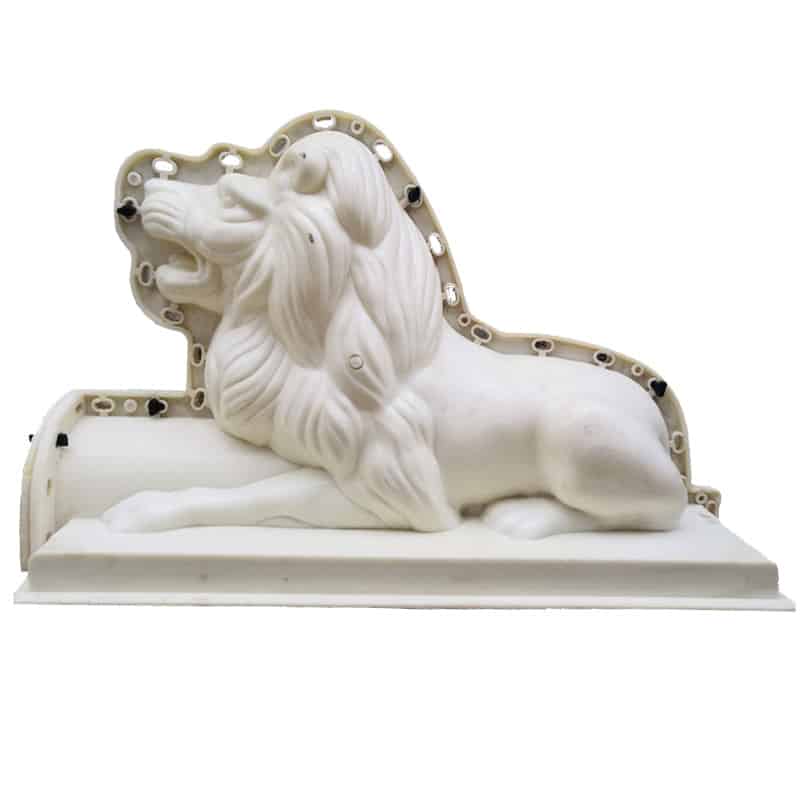The image depicts a white plastic mold of a lion, positioned on a white rectangular base. The lion is intricately detailed, featuring its mane and eyes, giving the impression that it is roaring. The lion's stance is small, similar to a souvenir item you might find in a shop. Around the edges of the mold, there are small holes, possibly designed for screws or other fasteners to secure the mold in place. Near the center of the lion, there is a cylindrical channel, suggesting it might be used to pump plastic or dye into the mold. The mold appears to be only one half, with the possibility of another half that could be sandwiched to complete it. Additionally, there is gray plastic framing that loops around the lion's head and down its back, featuring oval shapes that are either filled in or open. The lion is facing to the left, and the background is entirely white, enhancing the monochromatic aesthetic of the scene.